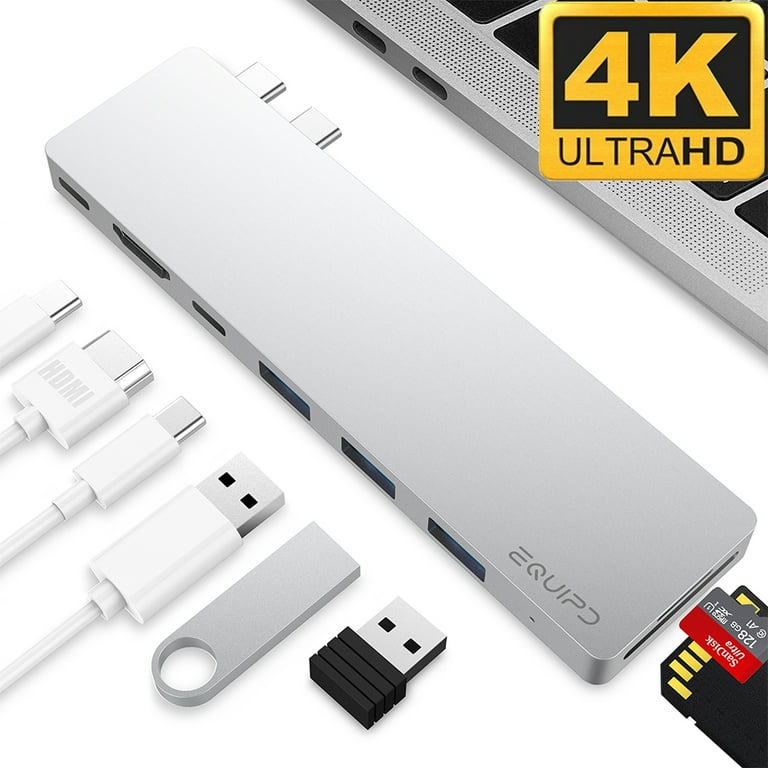The image is a meticulous close-up of a USB hub and various connectors arranged against a white background, resembling a product showcase or catalog display. The central element, a rectangular USB hub, features six extension ports prominently facing the viewer. This hub is primarily white with a sleek, steel-gray finish and has "EQIP" inscribed in dark silver lettering. Affiliated wires and connectors, including USB cables, HDMI slots, and SD card slots, are depicted both connected to and detached from the hub. To the bottom right, an assortment of USB sticks and wires, some black and silver, others white, are visible despite being partially cut off by the image's edge.

An upside-down red and white SanDisk SD card can be seen near the right side of the hub, enhancing the display's range of connectivity options. In the upper right corner, a laptop with a silver frame is partially cropped out, revealing a few black keys and two additional USB ports. Adjacent to this laptop corner, a yellow box with black accents displays the "4K Ultra HD" logo, underscoring the high-definition compatibility of the equipment. The minimalistic, white background emphasizes the electronics' design and functionality.